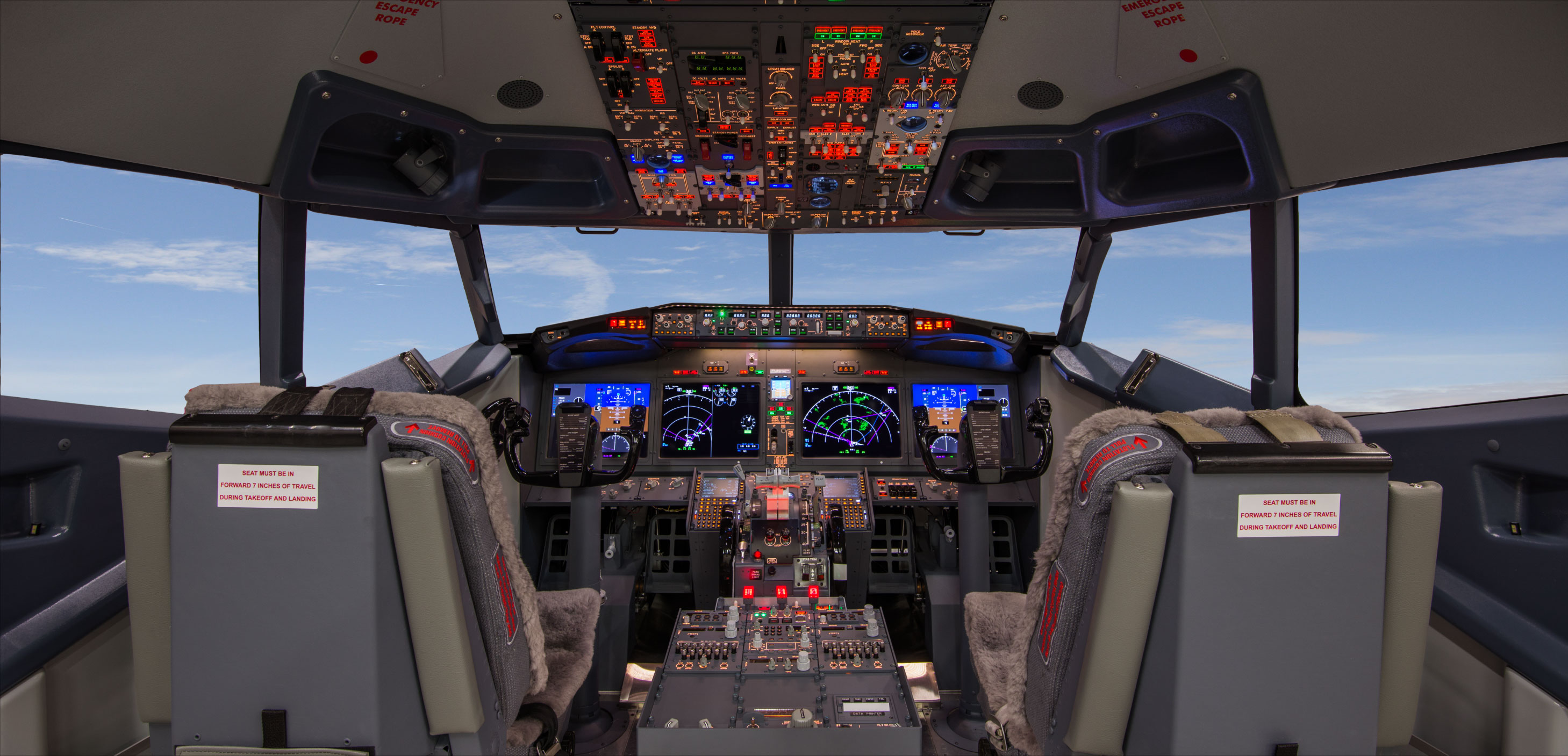The image showcases the cockpit interior of a commercial airliner. It features two empty seats, the pilot's and the co-pilot's, both equipped with yokes (steering wheels) and an array of navigation screens displaying radar and other flight information. The seats are olive and gray with harnesses draping over the headrests, and have white stickers with red text on their backs. The cockpit is brightly lit with numerous illuminated buttons, knobs, and gauges in various colors including red, green, blue, and black. The central instrument panel boasts about four screens, accompanied by additional buttons and switches above and below. The cockpit windows reveal a clear, blue sky outside, further enhancing the idea that this might be a simulation rather than an actual in-flight scenario. Several light indicators and levers adorn the overhead and lower panels, creating a vivid and detailed aviation environment.